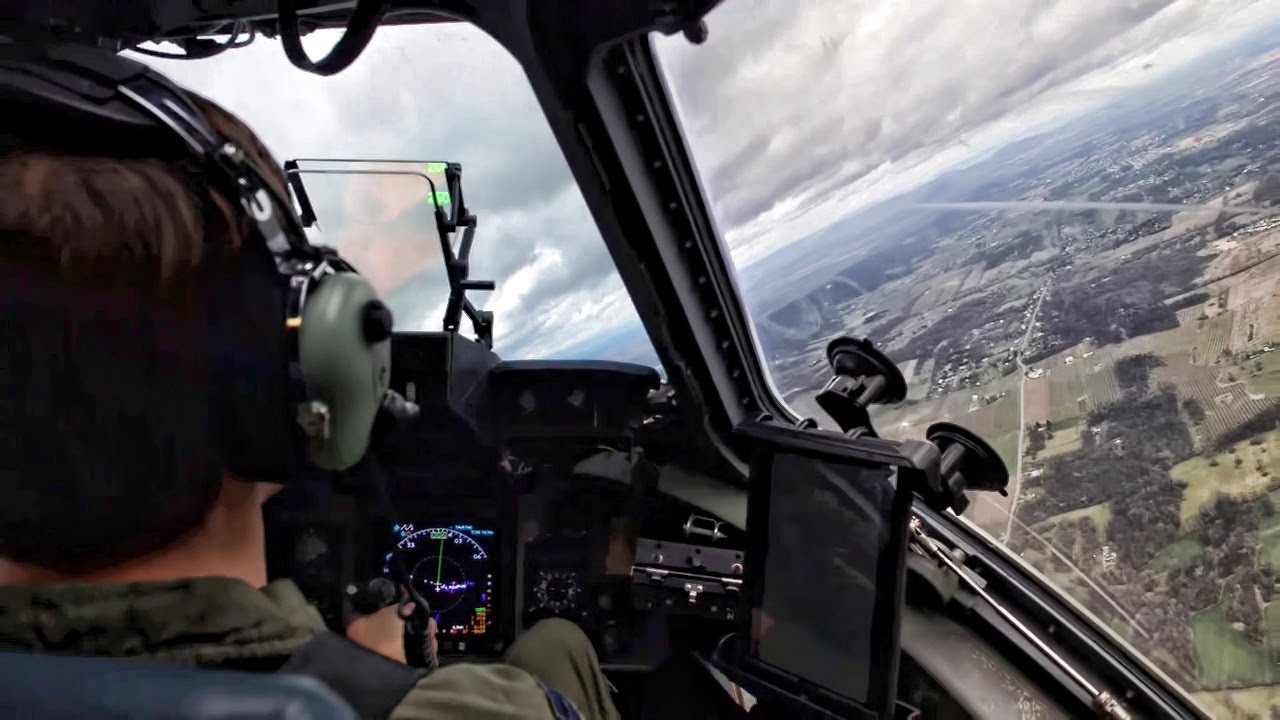The photo captures a detailed and immersive view inside the cockpit of a helicopter, with the pilot situated prominently on the right side. The pilot, who has short brown hair and is wearing green pants, is focused ahead with one hand firmly grasping the yoke in the middle of his seat. He is equipped with headphones, possibly engaged in communication with a navigator. Various instruments and displays, including a radar system, adorn the console before him, and an interesting display projects text into the air. To his side, a tablet is suction-cupped to the right, although it appears to be turned off. Through the cockpit windows, the helicopter flies over a patchwork of farmland, interspersed with trees and distant cities, beneath a cloudy sky. The scene is composed of a rural, farming area, approximately a few hundred feet below, adding to the serene yet dynamic nature of the flight.